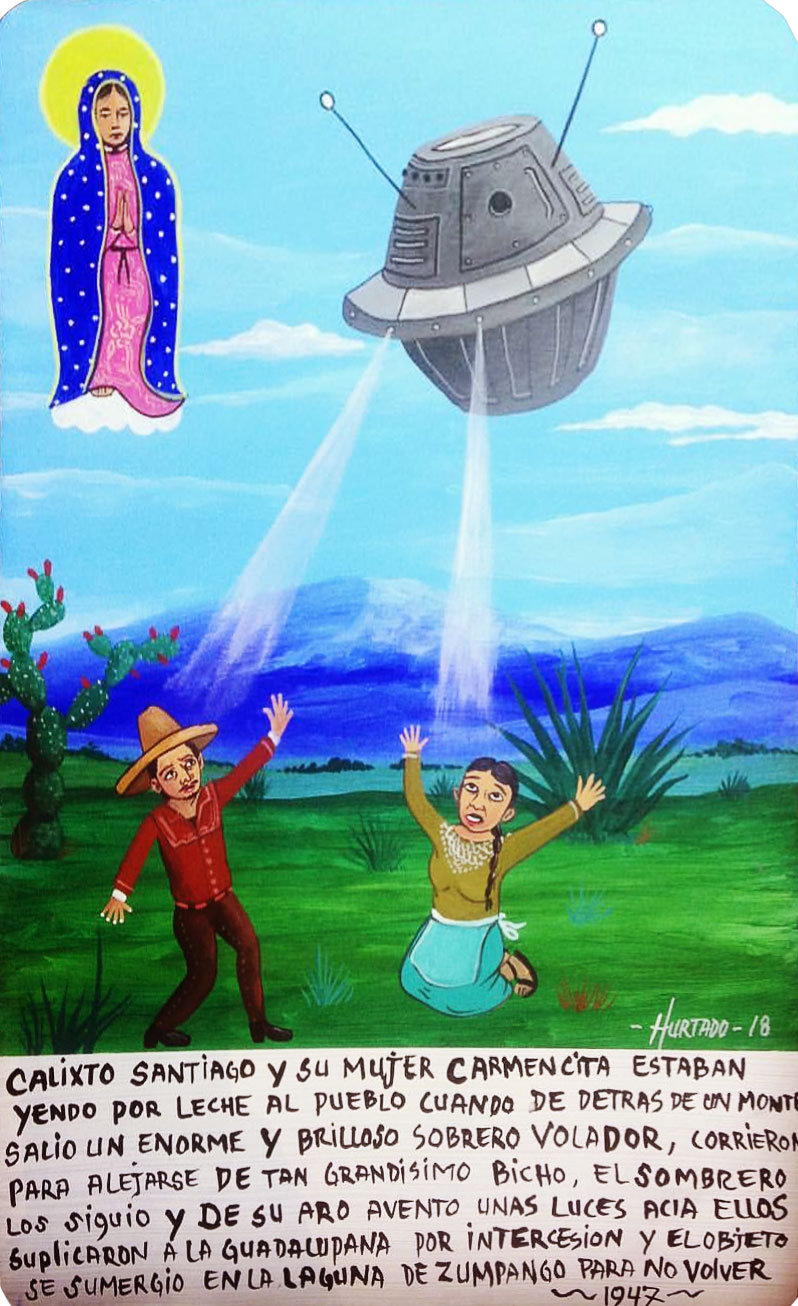The image appears to be a piece of folk art from 1947, created by an artist named Hurtado. It features a religious and somewhat surreal scene set in a green, mountainous area with very few clouds in the sky. In the top left corner, the Virgin Mary is depicted in a blue star-studded shroud with her hands folded in prayer, floating above a cloud with the sun behind her. To her right, there is a gray, industrial-looking spaceship with black and white-tipped antennae, beaming light down from the sky. Below, on the left, a man in a yellow sombrero, red shirt, and brown pants is standing and almost waving at the spaceship. On the right, a woman kneeling on the ground in a yellow ochre shirt and blue skirt raises her arms toward the mysterious light. The landscape around them features a cactus on the left and an aloe plant on the right, with blue mountains and a river in the background. The picture includes handwritten text in Spanish, suggesting a narrative element, although the specific details remain unclear. The overall scene blends traditional religious iconography with elements of science fiction, creating a unique, illustrative composition.